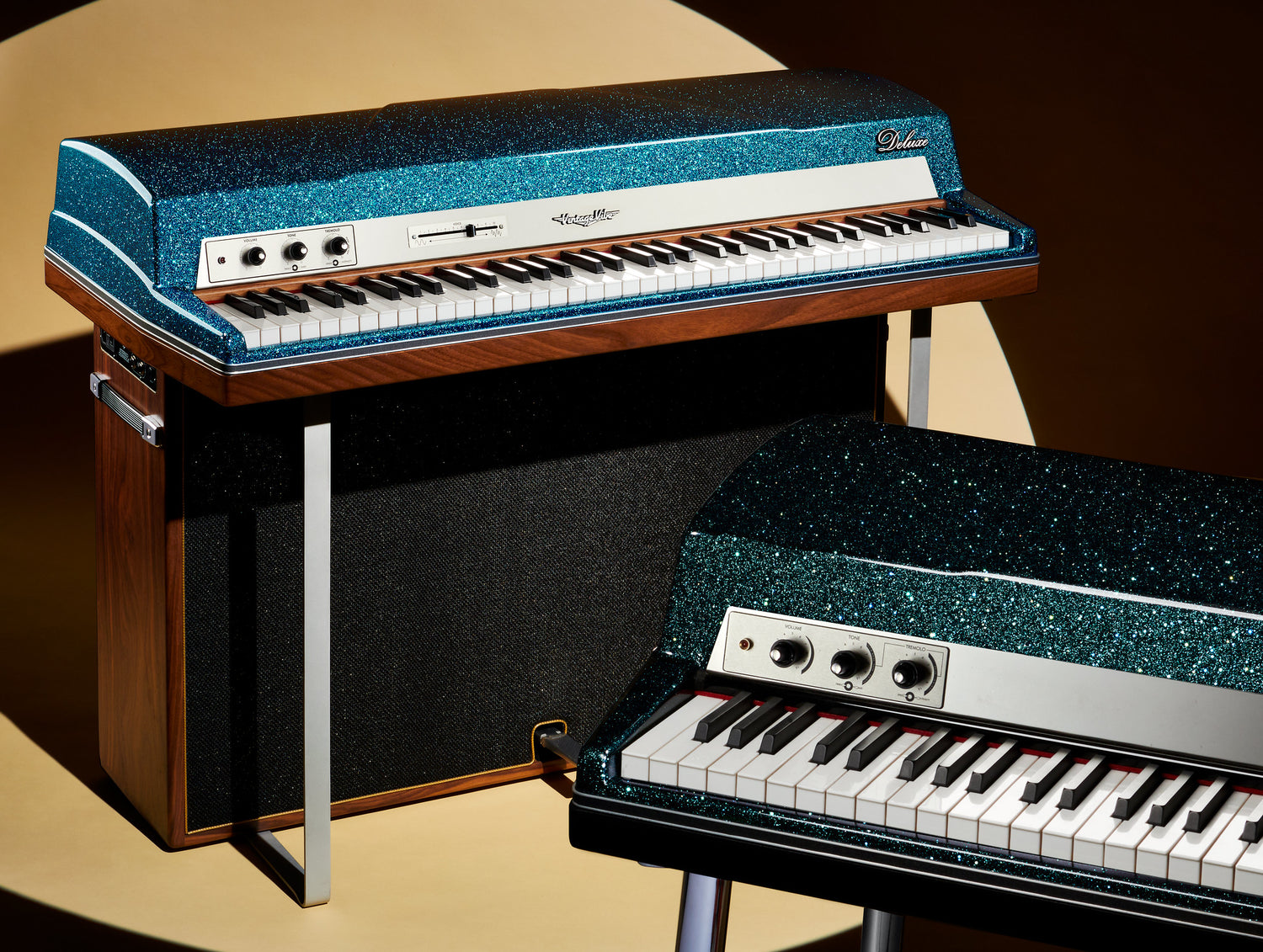The photograph features two vintage-style electric keyboards set against a dark background with a beige highlight on the left-hand portion. The primary keyboard on the left is encased in a large reddish-brown wooden frame with a black felt speaker cover. On top of this, a horizontal reddish-brown box supports a keyboard surrounded by a bright blue speckled panel. The white and black keys are prominent on this keyboard's right side, while a contrasting matte metal board above features three black dials on the left and a black slider just to their right. Centered on this metal board is a metal logo, and in the top right corner of the blue speckled portion, it reads "Deluxe."

To the right, an identical keyboard peeks into the frame, displaying a darker speckled blue surround. This keyboard is missing the black slider present on the primary one. Both keyboards exhibit shimmering, glittery colors reminiscent of space or futuristic aesthetics, with one leaning towards a teal or greenish hue, and the other appearing more blue and sparkly. The elegant, vintage design elements such as wood grain accents and the high-gloss speckled finishes give the keyboards a distinct and visually striking appearance, enhancing the sense of retro-modern charm.